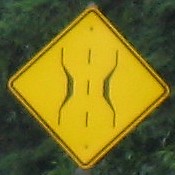The image features a square design set against a lush, verdant background filled with dense green trees and foliage. Prominently displayed amidst the greenery is a diamond-shaped highway sign. The sign is primarily yellow, bordered with a black outline, and has three black dashed lines running vertically down its center, creating a visually striking contrast against the lush backdrop. The vibrant green leaves envelop the sign, providing a vivid and lively context that enhances the prominence of the sign's design and its placement within the natural setting.